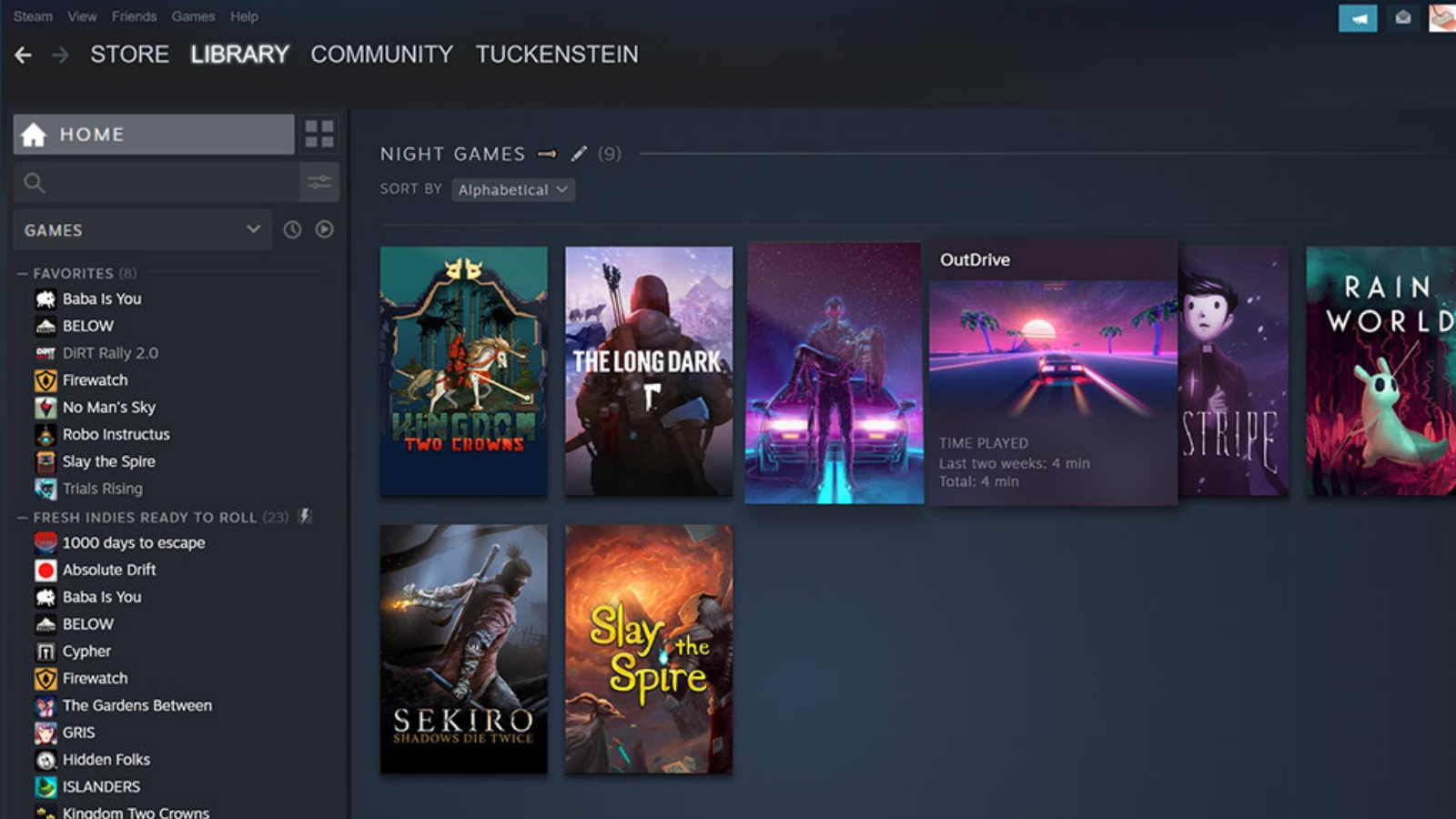This image showcases a user interface of a website or digital store, presumably named "T-u-c-k-e-n-s-t-e-i-n," that could be related to games or a community platform. The design features a sleek, black background accented with gray navigation links at the top, labeled: "Steam," "View," "Friends," "Games," and "Help." 

In the upper right corner, there is a teal-colored button with a backward-pointing arrow, an icon resembling an envelope on a black button, and another button with a white background displaying an icon that resembles a broom.

On the left sidebar, there is a "Home" button highlighted with a gray background and white font, accompanied by a home icon. Below it lies a search field characterized by a black input area and a gray magnifying glass icon, with a "Games" drop-down menu in black, displaying the text "Games" in white with a pull-down icon. 

Continuing down the sidebar, there is a section labeled "Favorites" followed by the number 8 in parentheses, indicating the user’s top picks. The list under "Favorites" includes the following games:
- Baba Is You
- Below
- Dirt Rally 2.0
- Firewatch
- No Man's Sky
- Robo Instructus
- Slay the Spire
- Trials Rising

There is also a segment titled "Fresh Indies," likely showcasing new independent games.